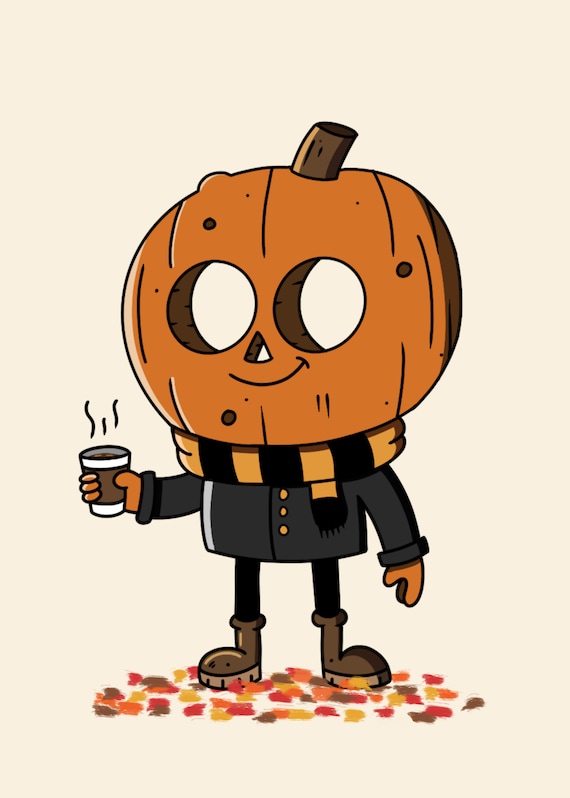The image portrays a whimsical, Halloween-themed scene featuring a character with a carved pumpkin head, complete with circular eyes, a triangle nose, and a black marker-drawn smile. This pumpkin-headed figure is digitally rendered in a comic book style, standing against a cream-colored backdrop. The character is dressed warmly in an orange and black scarf, a dark gray sweater, and brown boots, and it holds a steaming cup, suggesting it might be coffee or hot chocolate. Autumn leaves in vibrant shades of yellow, red, brown, and orange surround the figure, some even floating above its pumpkin head with a stem, adding to the festive atmosphere. The character also wears orange mittens and looks like an adorable, two-legged pumpkin man, ideally suited as a charming Halloween decoration.